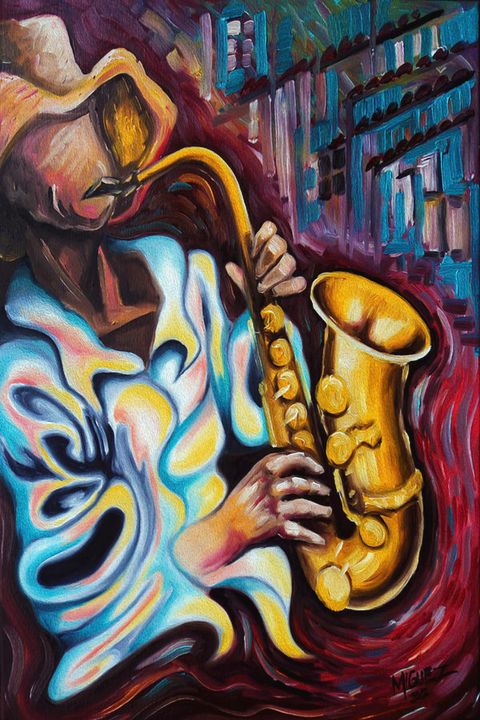This is a vibrant oil painting of a black man playing a brass-colored saxophone, centered against a red background with a blue building featuring glass windows and a black roof design. The man, depicted with a hand-painted texture, is adorned in a white, flowy shirt with hints of blue, yellow, and orange shades. His tan hands are seen firmly grasping the saxophone, with fingers positioned on both the top and bottom keys. The painting, rich in color and detail, also includes the man wearing a cowboy hat and is oriented to showcase the figure from the top of his hat to the bottom of his torso, creating a dynamic and engaging focal point.